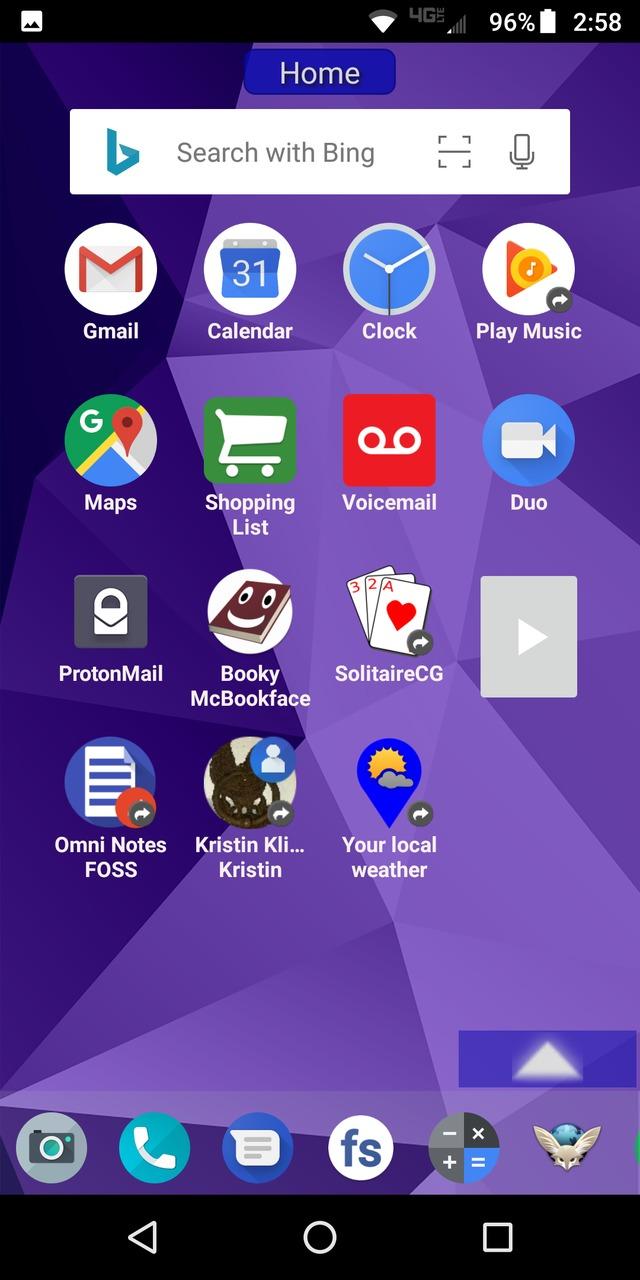The image appears to be a screenshot of a person's cellphone home screen. At the very top of the screen is a black status bar displaying various indicators: a notification for the gallery app, a 3-out-of-4 bar WiFi signal, 4G LTE connectivity with barely any service (only the first bar is white), a battery level of 96%, and the time displayed as 2:58. Below the status bar, a small blue box centered at the top bears the word "Home" in white text.

Directly beneath this blue "Home" indicator, there is a Bing search widget. The widget features a white search box with a blue Bing logo (a stylized "B") and offers options for QR scanning, barcode scanning, and voice search. The wallpaper of the home screen is a purple kaleidoscopic pattern comprising various shades of purple.

The home screen displays numerous app icons, including Gmail, Calendar, Clock, Play Music, Maps, Shopping List, Voicemail, Duo, ProtonMail, Bookly, MacBook Face, Solitaire, DVD, Omni Notes, FOSS, your local weather, and an app labeled "Kristen something." There is also a mysterious white square icon with a right triangle in the middle.

At the bottom of the screen, the user has placed their primary apps: Camera, Phone, Text Messages, an app labeled "FS," Calculator, and an enigmatic app featuring an icon that resembles a winged rabbit. The overall look of the screen suggests that it might be an older version of the operating system, given the dated design of the icons.